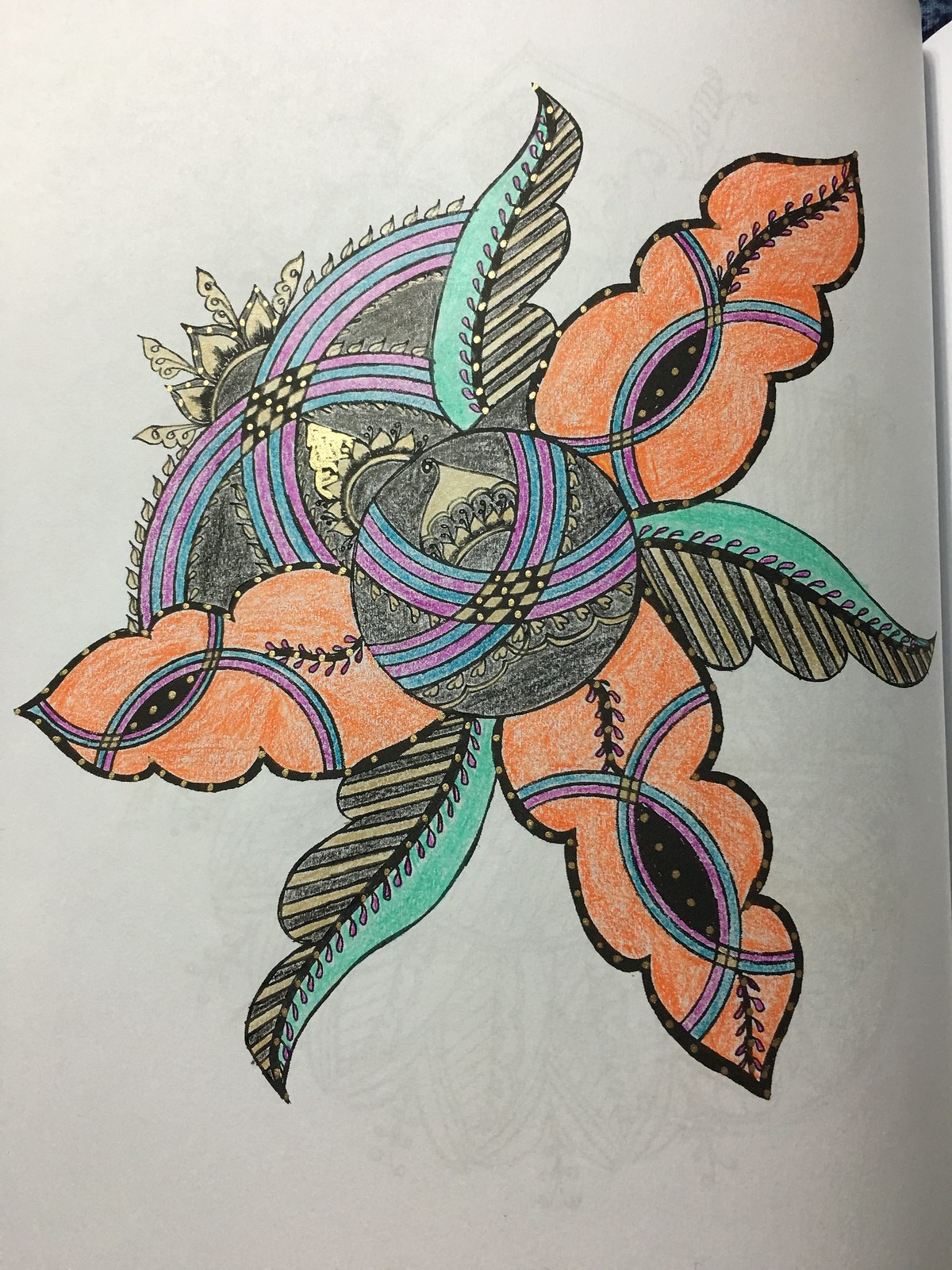This detailed artwork is an abstract rendition of a flower on a white piece of paper, created likely with pencils or crayons. At its core, there's a black circle decorated with small semi-circles, outlined in gold and filled in with a light gray and black. Two hearts are embedded within these semi-circles. Above the central circle, a Hershey Kiss-shaped figure, colored tan, is flanked by small, black teardrop shapes accented with gray.

Radiating out from this center, to the left and right, are diagonal crisscrossing lines in alternating purple and blue colors. At their intersection, a checkerboard pattern in tan and black emerges, with tan circles embellishing the black squares.

Surrounding this central motif are several large, orange leaf-like shapes, each featuring similar crisscrossing lines in purple and blue, reminiscent of rainbows. These leaves are embedded within wider leaves that are half teal green with small purple circles and half black with diagonal gold lines. Further embellishing the composition, a crown-like shape with tan swirls appears in the upper left, resembling the leaves of a plant with black edges and tan dots.

Additional design elements include pea pod-shaped figures with black interiors and gold dots, and multiple wavy leaves in sets of three, alternately colored in black and gold, as well as orange. This meticulous and vibrant design captures the viewer’s attention with its intricate patterns and harmonious color scheme.